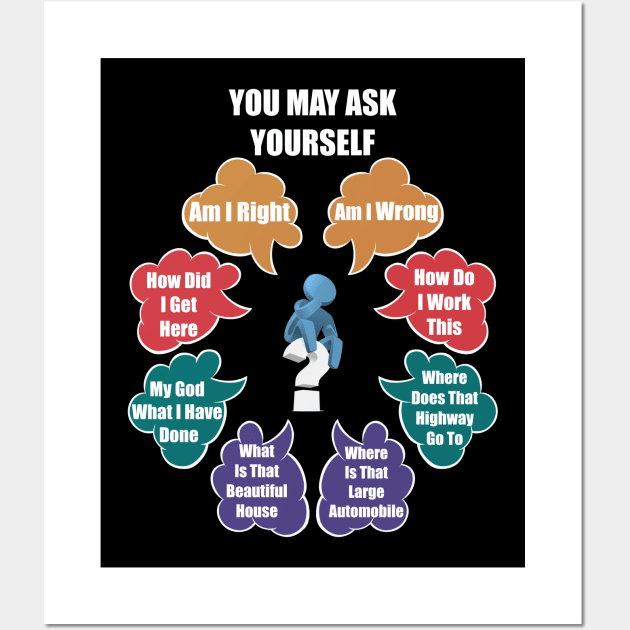This poster features a striking black background with a prominent white border against a light beige wall. Central to the design is the phrase "You may ask yourself" written in thick white font. Surrounding a blue stick figure seated on a 3D white question mark, numerous colorful thought bubbles capture a series of reflective questions: "Am I wrong?", "How do I work this?", "Where does that highway go to?", "Where is that large automobile?", "What is that beautiful house?", "My God, what have I done?", "How did I get here?", and "Am I right?". The thought bubbles are colored yellow, red, green, and blue, and each contains white text. This setup suggests an introspective theme, possibly inspired by lyrics from a Talking Heads song, with the thought bubbles pointing towards the stick figure in the center, highlighting its sense of contemplation and self-inquiry.